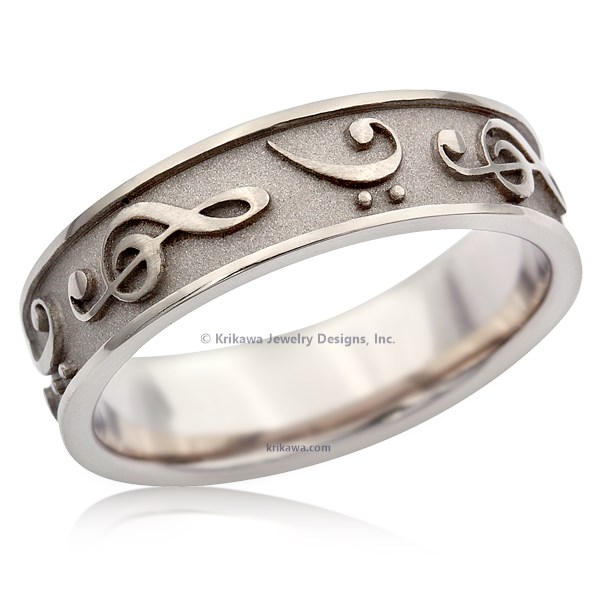This close-up image captures a silver band ring against a plain white background. The ring is positioned at an angle, with the right side tilted upward toward the upper right corner, creating a subtle shadow or reflective effect below. The exterior of the band features raised musical notes, including a treble clef, which are carved into the silver. These symbols are set against a darker, rougher pewter-colored background that contrasts with the shiny, raised edges and smooth plain interior. In the center of the image, small light gray text reads, "© Krikawa Jewelry Designs, Inc." Below this, in even finer print, is the website "krikawa.com".